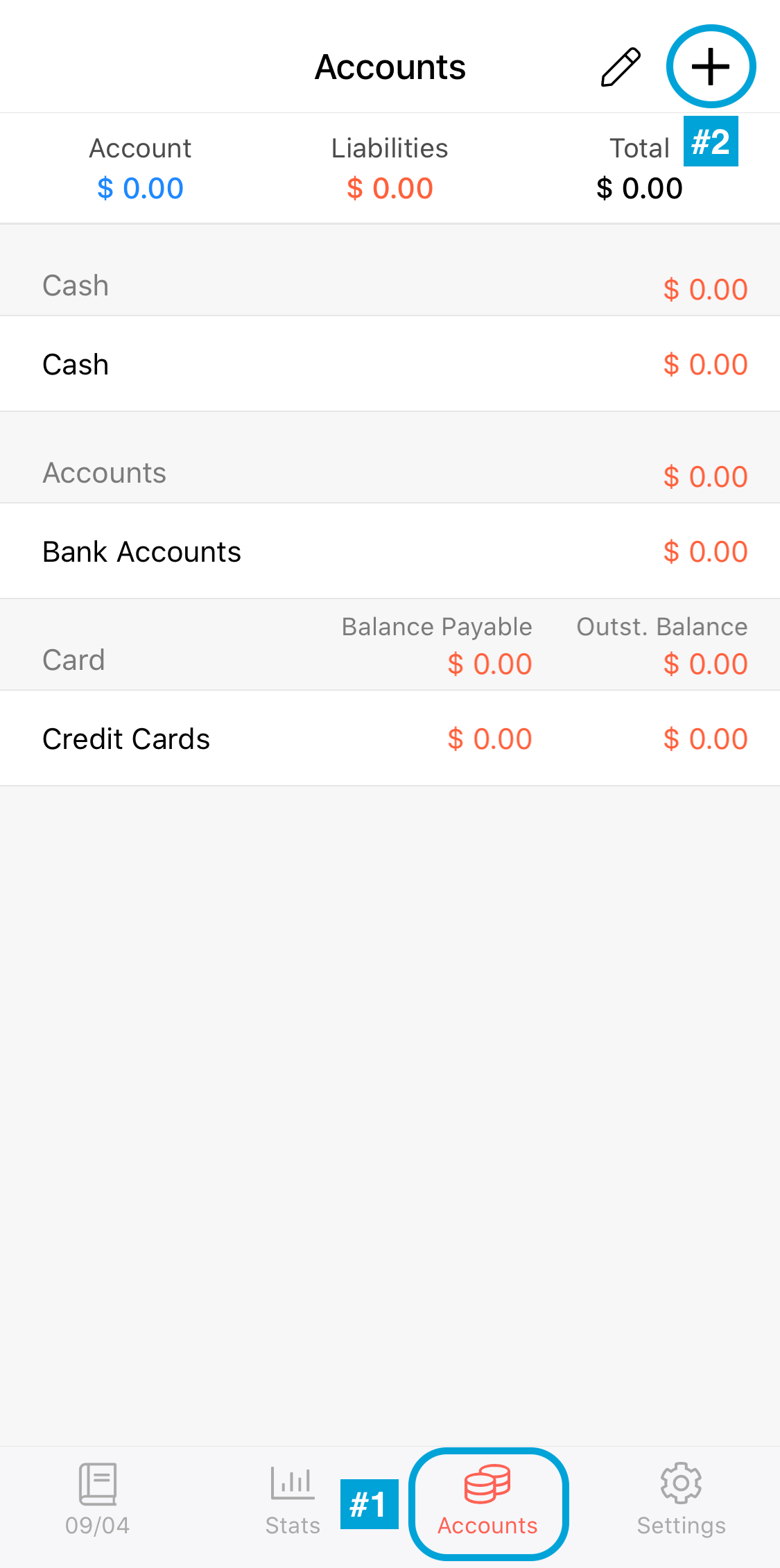A detailed screenshot from a mobile application interface is displayed. At the center top in bold black text, the word "Accounts" is prominently featured. To the right of this, there is an icon of a pencil and a plus sign encircled in blue, signifying options for editing or adding accounts. Below this, a line separates the header from the detailed sections.

The main section is divided into three evenly spaced columns. The left column, labeled "Account" in black text, has a dollar sign followed by "0.00" beneath it. The middle column is labeled "Liability" in black text, showing an amount of "0.00" in orange. The right column, titled "Total" in black, also shows "$0.00" in black. Adjacent to the "Total" label, a small blue box contains a white pound sign and the number two. Another line separates this section from the subsequent content.

The next section features a large gray rectangle with the label "Cash" and an amount of "0.00" in red text. Immediately beneath it, a white box also labeled "Cash" and showing "0.00." Other gray boxes labeled "Accounts," "Bank Accounts," and "Card" also display "0.00" beneath them. Within these boxes, additional text on the left-hand side reads, "Balance Payable" and "Outstanding Balance," both showing "0.00." Under the "Credit Card" label in another white box, "0.00" is displayed.

At the bottom of the screen, there are four tabs, each featuring different labels: "0904," "Stats," "Accounts," and "Settings," indicating different sections or functionalities of the app.